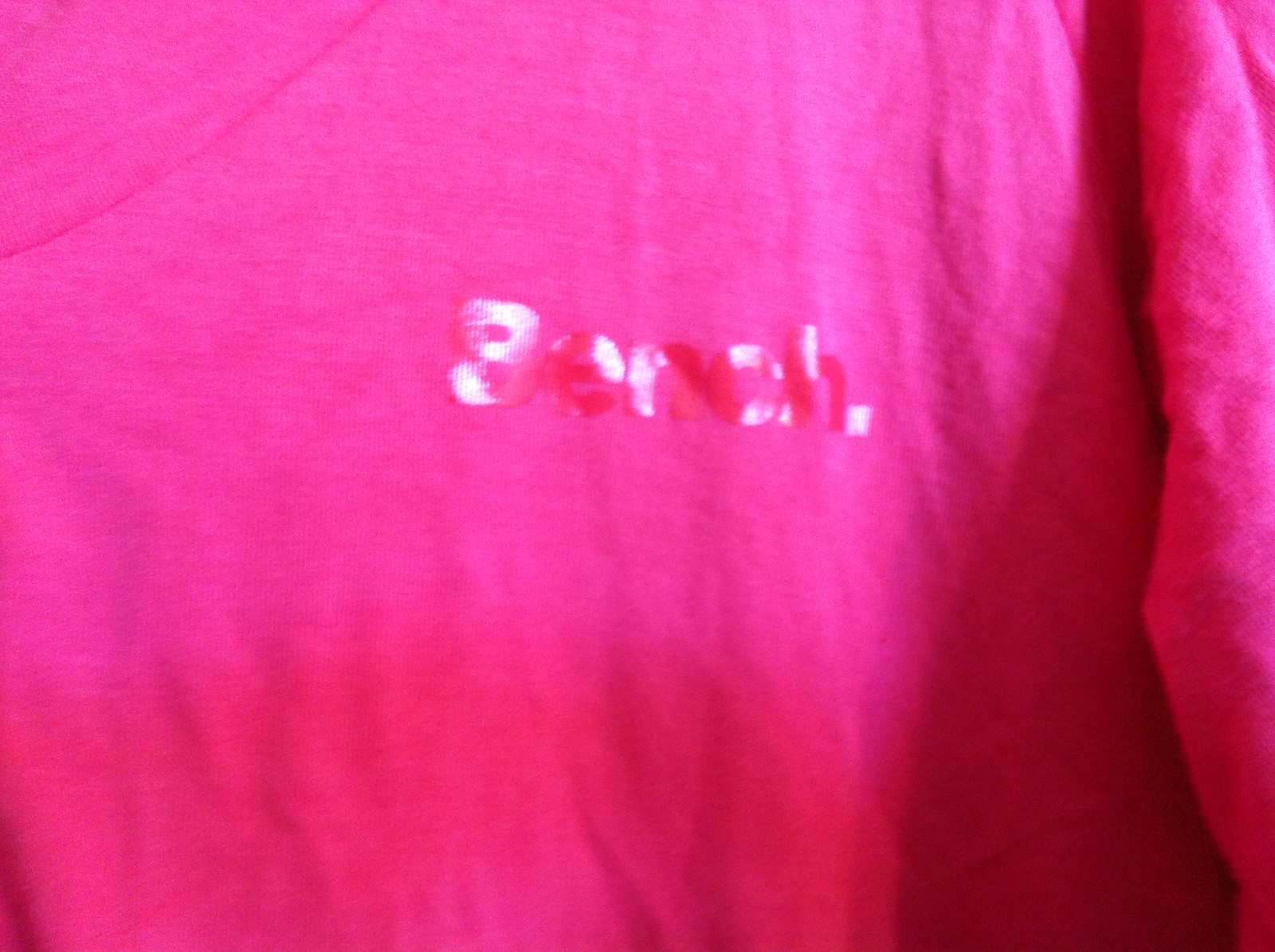This is a photographic image of a knit long-sleeve t-shirt, displayed in a landscape orientation within a rectangular frame. The shirt, occupying the entire frame, features a prominent logo at the center. The logo reads 'Bench.' in capitalized letters, followed by a small square resembling a period. The word 'Bench.' appears to be either screen-printed or made from a shiny two-tone material, possibly blending white and hot pink hues. There is a notable shadow on the right-hand side, likely caused by the sleeve overlapping part of the garment, adding depth to the image.